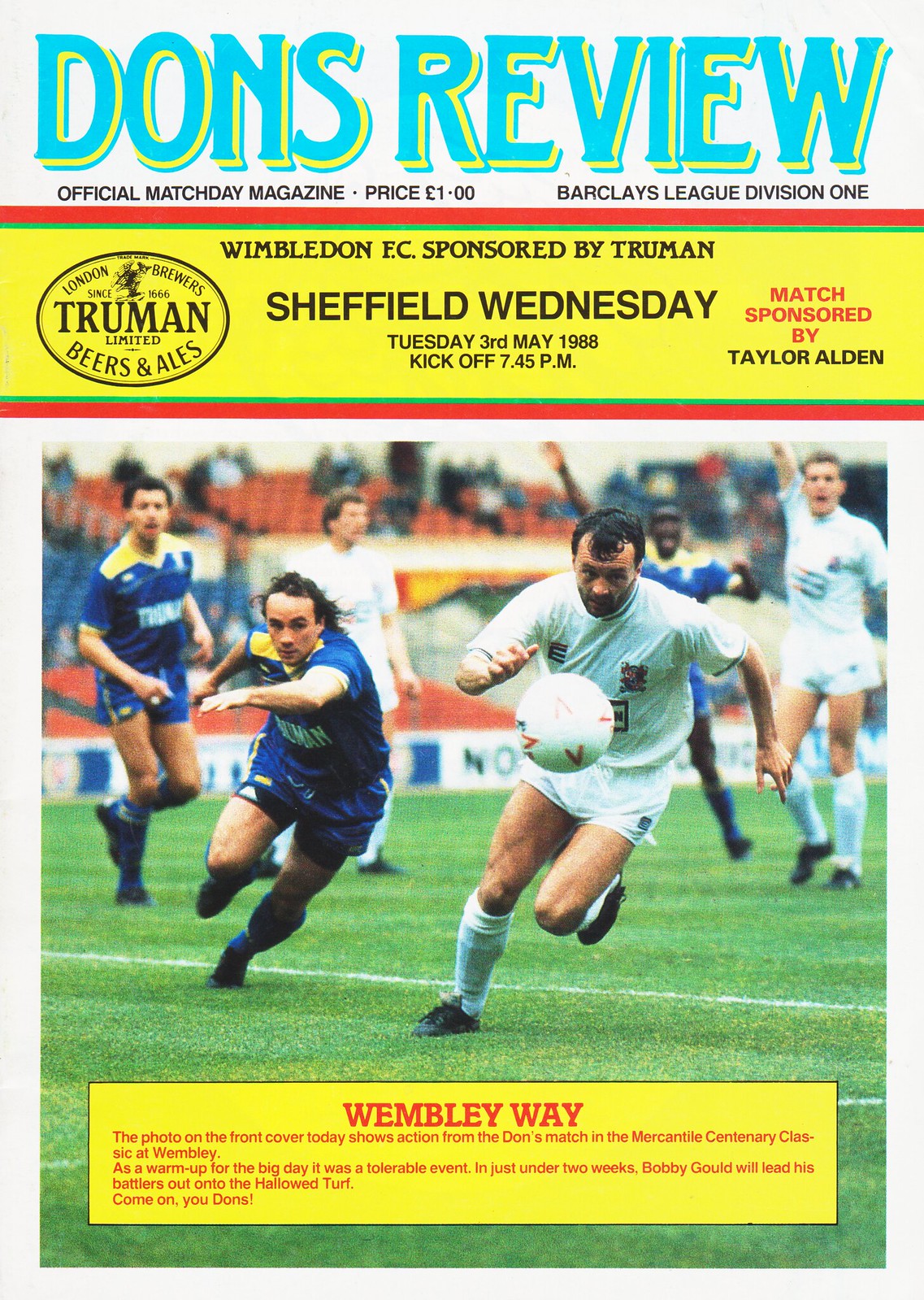The cover of this vertically aligned soccer program, titled "Don's Review," is dominated by a light gray background with bold, all-caps blue letters outlined in yellow. It prominently displays, "OFFICIAL MATCH DAY MAGAZINE PRICE £1.00." On the right, "Barclays League Division 1" adds context. 

At the top, a horizontal white stripe announces that the Sheffield Wednesday match is a Wimbledon-sponsored event scheduled to kick off on Tuesday, 3rd May 1988, at 7.45 p.m. Below this, a yellow banner with red horizontal stripes provides further text, mentioning "Wimbledon FC Sponsored by Truman," and noting the match sponsor, Taylor Alden.

The lower half of the cover is occupied by an action photograph from a soccer match. The scene captures the dynamism of the sport with players on a green turf field lined with white markers. The stands in the blurred background feature seated spectators, interspersed with red and blue seats. Prominently, the image shows two soccer players in blue uniforms with yellow shoulder details, and another in a white kit, all actively engaging with the ball. Additional blurred figures add depth and motion to the scene.

At the bottom, a yellow box with red text titled "Wembley Way" credits the photograph and notes it was taken at a Dons match in the Mercantile Century Classic at Wembley. It highlights the anticipation surrounding this warm-up event, leading to the significant upcoming match where Bobby Gould will guide his team onto the revered Wembley turf.